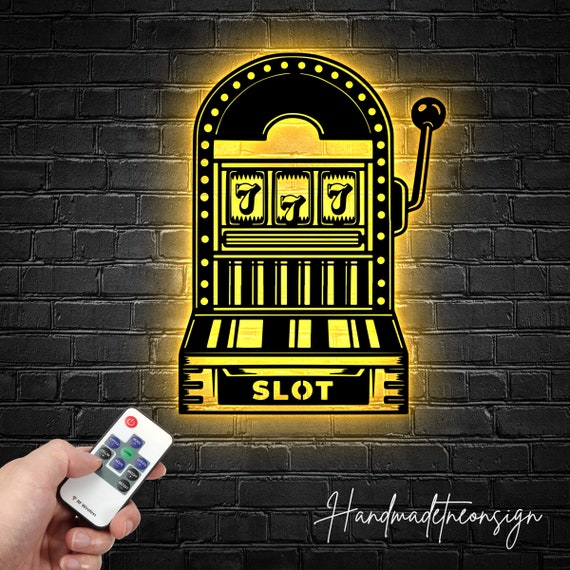The image features a computer-generated, square slot machine prominently displayed in the center against a realistic brown brick wall background. The slot machine is black and yellow with a lever on the right side and the numbers "777" illuminated across the display, signifying a jackpot. At the bottom of the slot machine, the word "SLOT" is written in all capital letters. In the lower-left corner of the image, a man's left hand is holding a sleek, silver remote control with blue, black, red, and green buttons. In the lower-right corner, there is cursive text that reads "HANDMADE NEON SIGN" written as one word. The hand and remote appear real, contrasting with the digitally created slot machine and background.